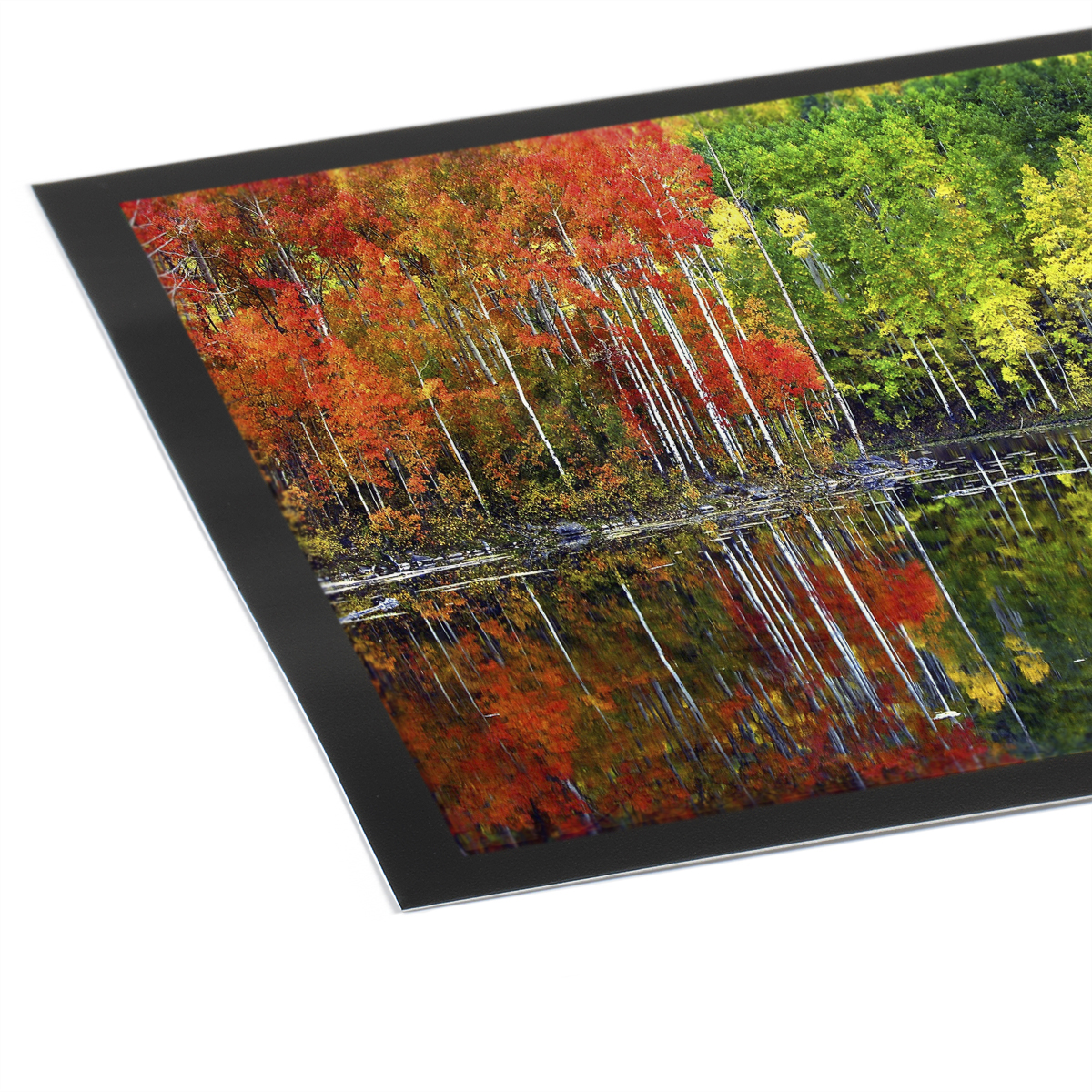This color photograph, set against a white backdrop and outlined with a thick black border, captures a striking, diagonal composition where a significant portion of the image seems to be off-screen, tilted upwards to the right. The scene within the photograph is divided distinctly between two seasons: the left side showcases a serene grove of birch trees with their white trunks surrounded by vibrant autumn foliage in hues of red, orange, and slightly yellowish-green. The foreground features a calm body of water that mirrors the stunning fall colors, though the reflection is slightly rippled, possibly due to a gentle breeze. Contrasting this, the right side of the photograph reveals the same grove in a different season, likely spring or summer, where the trees stand verdant with bright, varied shades of green. This section also includes a part of the water's reflection, capturing the lush greenery. The entire composition suggests a masterful blend of photography and art, creating an ethereal snapshot bridging two different seasonal landscapes within the same harmonious scene.